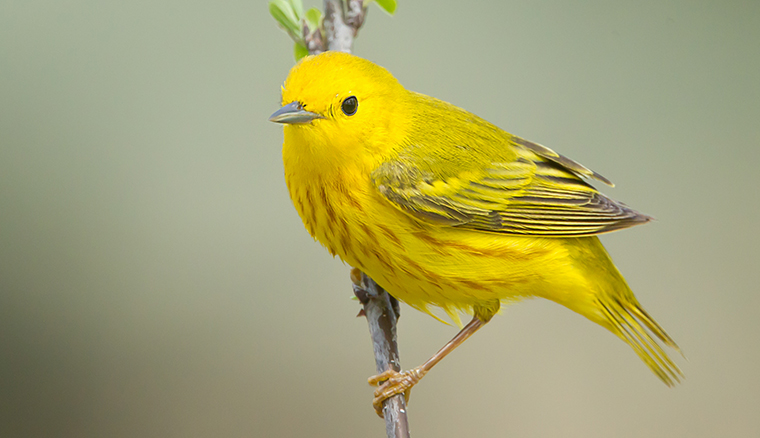An up-close photograph captures a vibrant yellow bird, likely a finch or a goldfinch, perched gracefully on a tree branch. The bird's body is predominantly a brilliant yellow, with subtle brown patches on its torso and darker yellow highlights mixed with some black on its wings. The wingtips exhibit a striking pattern of yellow and black stripes. It has a sharp beak that is a light gray-blue color and all-black eyes, exuding a keen, alert expression. The bird's legs and feet are a muted yellow, with a hint of bronze or copper hues. The branch it clings to is a mix of brown and white, extending from the bottom center to the top center of the image, with some small green sprouts emerging at the top. The background is a blurred, predominantly grayish tint with darker areas in the lower left and upper right corners, creating a soft, out-of-focus backdrop that highlights the bird's vivid colors.